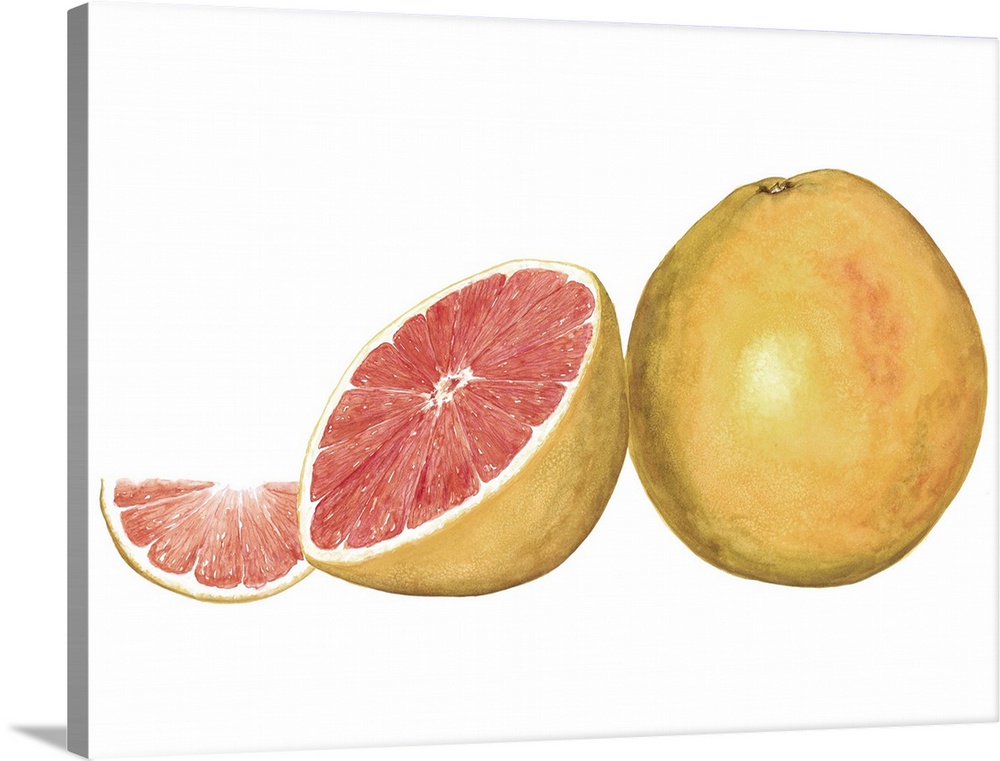This is a detailed color or AI-generated illustration presented in landscape orientation, featuring three renditions of a grapefruit against a white background. On the right, there is a whole grapefruit with a yellowish-orange peel that has subtle patches of brown and a distinctive top where the stem used to be. The grapefruit is shiny, suggesting a fresh, realistic appearance. In the center, propped slightly against the whole fruit and facing the upper left, is a grapefruit sliced in half, revealing a beautifully detailed interior with dark pink-reddish flesh, perfectly structured sections, a white central core, and a white rind. On the far left, there is a single grapefruit wedge, positioned so the juicy pink interior faces the viewer, showing off its eight meticulously rendered segments. This detailed illustration is printed on a canvas, which is propped on its longer side, and the edge of the canvas is a solid gray, enhancing the perceived depth of the artwork. The image does not wrap around the edges, emphasizing the contrast between the illustration and its white background.